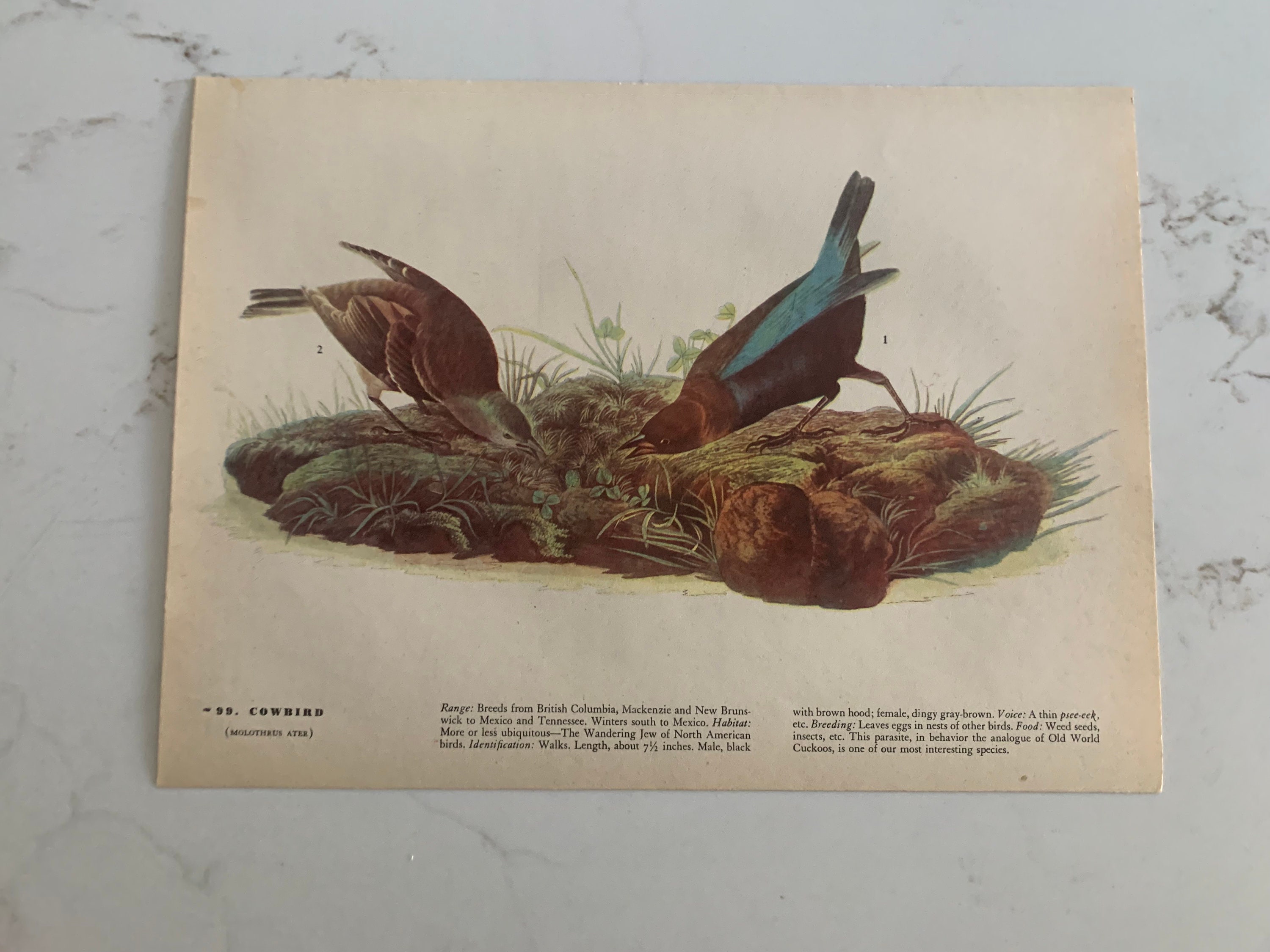The image is a detailed photograph of an illustration, likely an artistic plate from a book, magazine, or brochure. The background is a white marble-like countertop beneath a slightly yellowed sheet of paper, indicating age but not excessive wear. The illustration features two cowbirds standing on a bed of soil, rocks, and various vegetation including grass and clover. The birds are depicted with their heads bowed down, as if pecking for insects or interacting with each other. The male cowbird has a distinctive brown head, dark blackish body, and blue-tinted wings, while the female has a grayish head and a brown, less colorful body. At the bottom left of the illustration, the word "Cowbird" is inscribed. Additional text provides information about the cowbirds' range, breeding from locales such as Columbia, McKenzie, and New Brunswick to New Mexico and Tennessee, and notes their wintering extends south to Mexico. It also describes their habitat as ubiquitous, labeling them the "wandering Jew of North America birds."